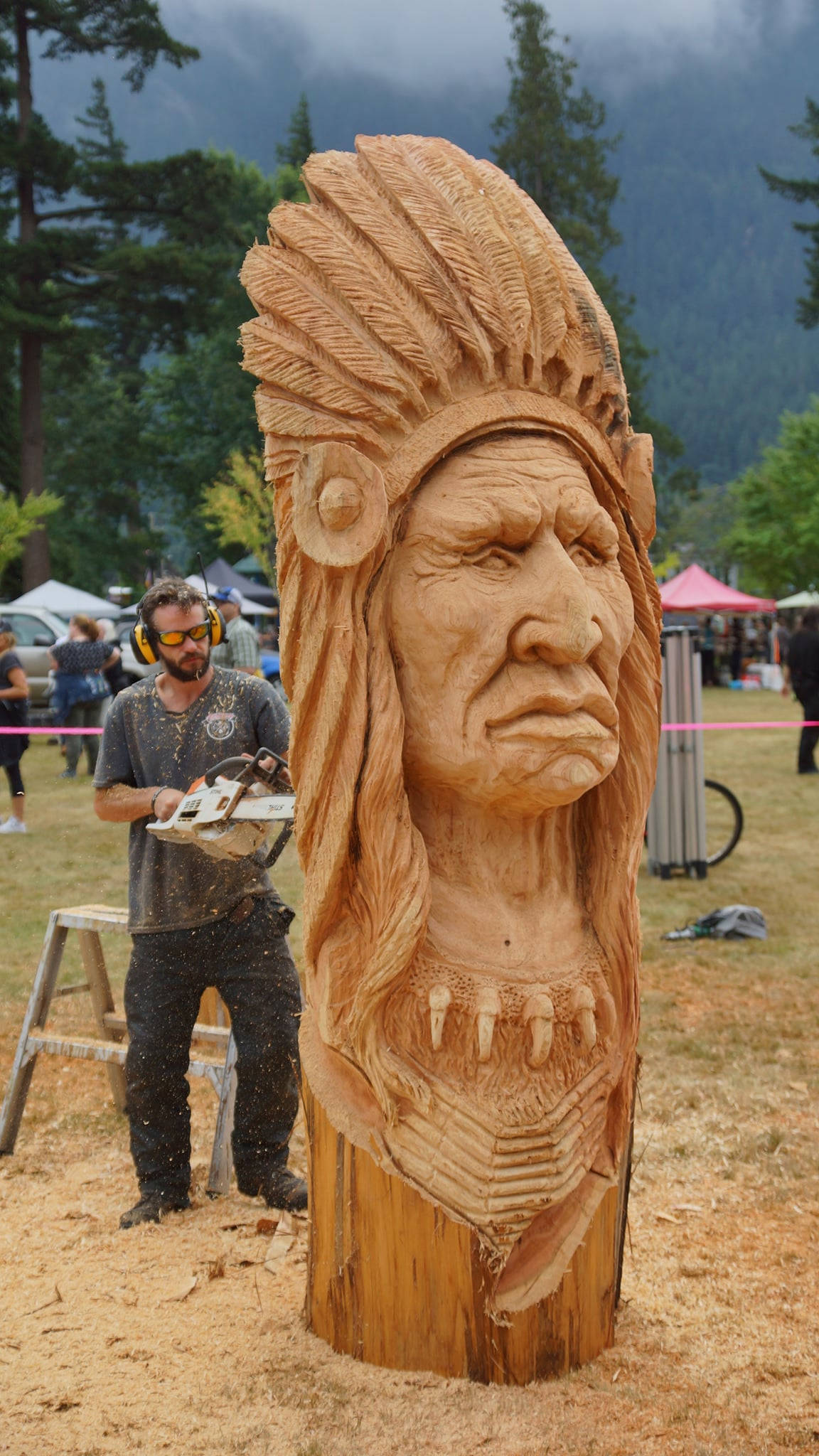The photograph captures an intricate scene centered around a substantial, eight-foot-high wooden statue of a Native American figure, characterized by a detailed feathered headdress, long hair, and an ornate tooth necklace. The statue, carved from a large log, features age lines giving it a venerable appearance and is positioned facing towards the right. A man, dressed in a gray shirt, black pants, and boots, stands behind the statue wielding a chainsaw deeply embedded in the wood, actively engaged in the carving process. He is equipped with protective goggles, reflective glasses, and headphones. Sawdust surrounds the base of the statue, indicating ongoing work. The background reveals a lively outdoor setting, possibly a festival, with numerous colored tents and canopies, people milling about, cars parked, and dense woods framing the scene.